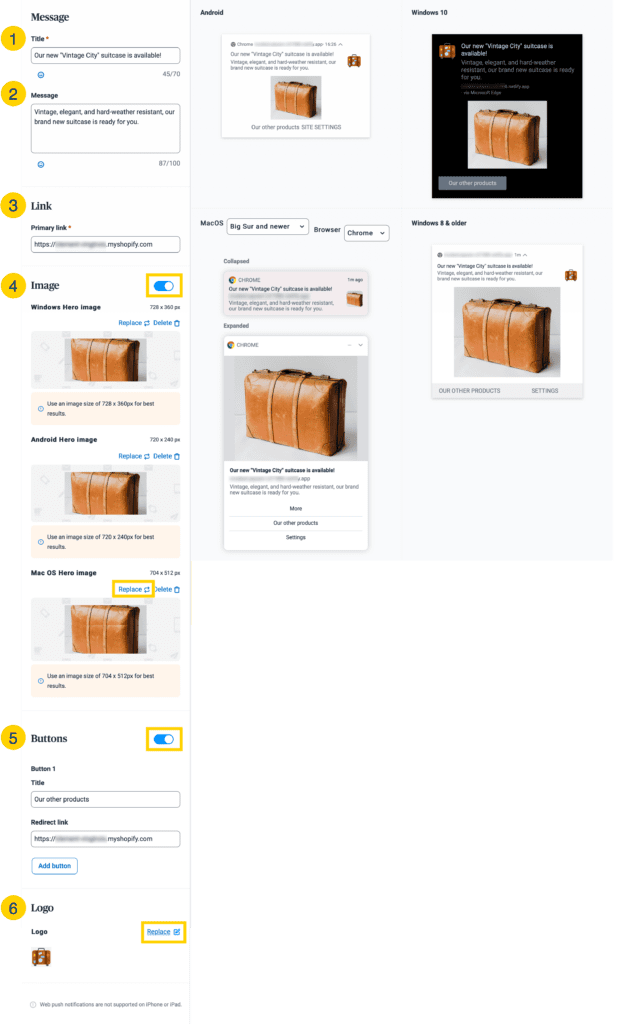**Detailed Caption for Image:**

The image features a white background with various elements arranged in a sequential and hierarchical layout. On the left side, there is a series of numbered points, each enclosed in a yellow circle. 

1. **Number 1**: Followed by a message box containing specific text (not specified).
2. **Number 2**: Accompanied by another message box with text.
3. **Number 3**: Marked by a link element within a yellow box.
4. **Number 4**: Denoted by an image inside a yellow box. Additionally, there's a small yellow square featuring a blue toggle button next to a picture that resembles a suitcase. Beneath this, there are very small blue words accompanied by another image of the same suitcase. Further down, there is yet another image of the suitcase enclosed within a yellow-bordered box.
5. **Number 5**: Labeled "Business," this section includes a yellow square with a blue toggle button inside, a search bar, another square, and a blue button.
6. **Number 6**: Titled "Logo," displaying multiple logos.

On the right side of the image:

- A large blue box with the word "Android," accompanied by descriptive text and multiple images of the suitcase.
- Farther to the right, there's a section labeled "Windows," featuring a black square with the suitcase image and a modem icon next to another black suitcase.

The detailed arrangement and color-coded elements guide the viewer through various messages, links, images, and interactive components on the page.